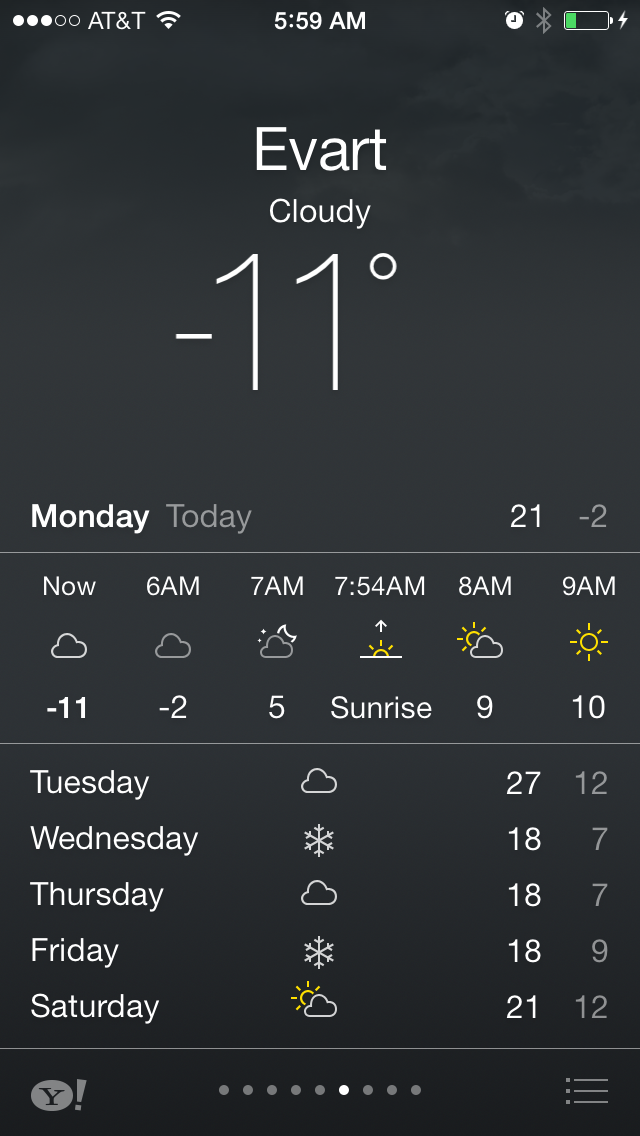The screenshot depicts a weather app displayed on a cell phone, specifically connected to the AT&T server, as indicated by the network information located at the top left of the screen. It is early morning, with the time shown as 5:59 AM in the status bar.

At the top of the screen, adjacent to the time, there is an icon showing the battery life. Below these indicators, the name of the location, "EVART" (in capital letters), is prominently displayed. Directly beneath the location name, the weather condition is specified as "Cloudy." The current temperature is a frigid minus 11 degrees Fahrenheit.

Further down, the app notes that it is Monday. This is followed by a section providing more details for the day. The word "Today" is displayed in gray color next to white text specifying additional details. To the right of this text, the high and low temperatures for the day are given as 21 degrees and minus 2 degrees Fahrenheit, respectively.

The hourly weather report follows. It begins with the current time ("Now"), and includes subsequent intervals at 6 AM, 7 AM, 7:54 AM (corresponding with sunrise), 8 AM, and 9 AM. For each listed time, the type of cloud cover is represented by various icons, with the corresponding temperature displayed beneath each icon.

The navigation continues to a broader forecast covering the upcoming days of the week. The days listed include Tuesday, Wednesday, Thursday, Friday, and Saturday. Each day has a weather icon representing the predicted conditions (cloudy, snowy, partly cloudy, etc.). The high and low temperatures for each day are also provided. Tuesday shows a high of 27 degrees and a low of 12 degrees. Wednesday, Thursday, and Friday each have highs of 18 degrees and lows of 7 degrees, with Friday slightly varying at 9 degrees. Saturday indicates a high of 21 degrees and a low of 12 degrees.

At the bottom of the screen, there is an underline followed by the Yahoo! logo, accompanied by an exclamation mark.